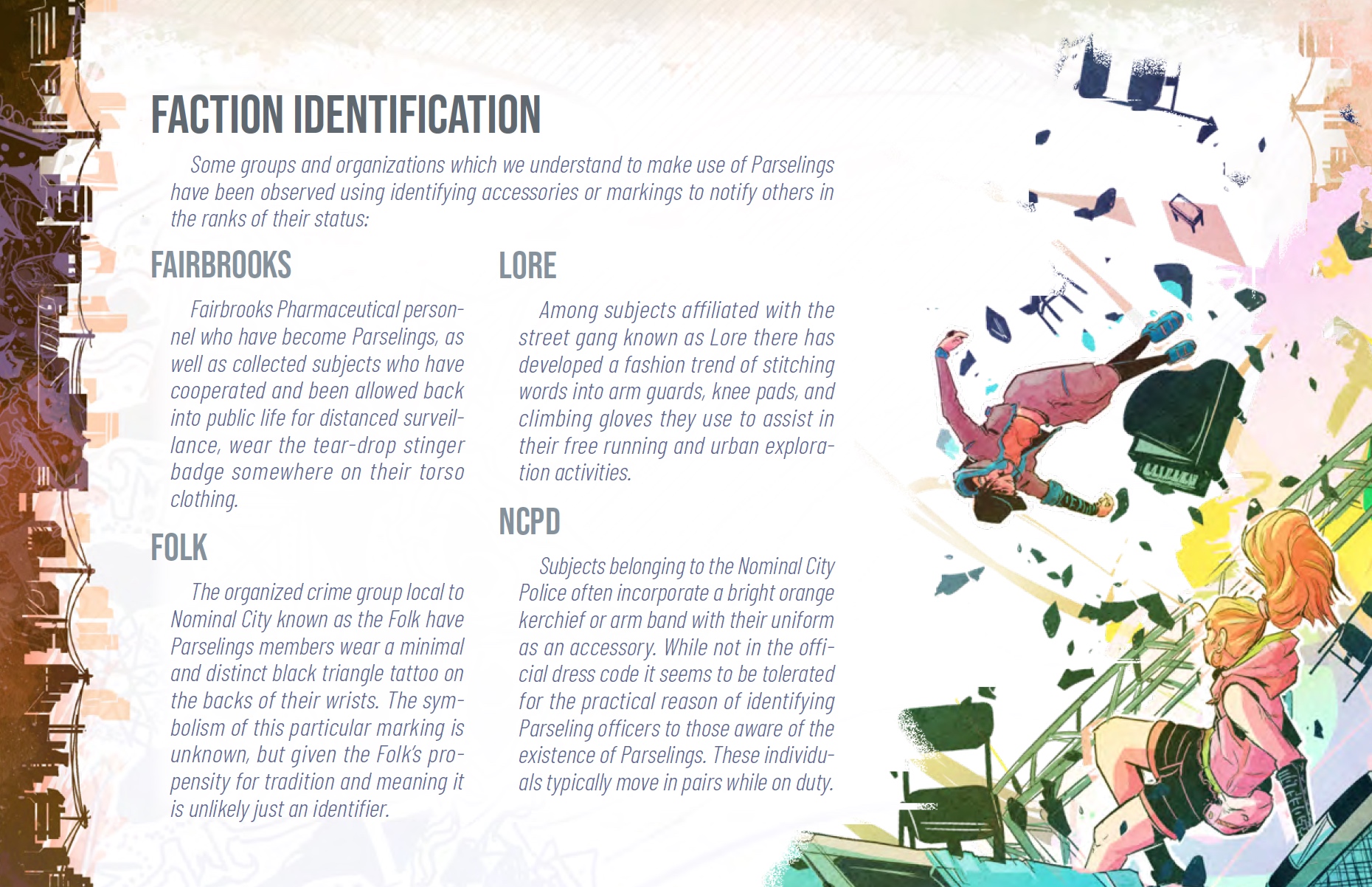The image is a detailed illustration featuring a chaotic scene on the right-hand side, where various objects and individuals are whirling through the air, suggesting a tumultuous event. Notably, there's a cartoon-like or comic book illustration of a piano flying through the air amidst geometrical shapes and a striking pink wave. Below the flying debris, which also includes parts of a metal tower or stadium seating and chairs, is a depiction of a girl with a high red ponytail, dressed in pink and black attire. 

The background includes a sideways city skyline, adding to the surreal and disorienting effect of the scene. Among the people being tossed around is a woman with blonde hair and another individual, possibly male, both seemingly caught in an explosion or a tornado-like vortex.

On the left side of the image is a block of text titled "Faction Identification," which lists four categories: Fairbrooks, Lore, Folk, and NCPD. Each category describes the identifying accessories or markings used by members of different groups, likely from a fantasy game or a similar narrative. Fairbrooks personnel, for instance, wear a teardrop stinger badge on their torso, while members of the Folk display a distinct black triangle tattoo on the backs of their wrists. The text elaborates on how these identifiers mark the status and affiliation of members within their respective factions.